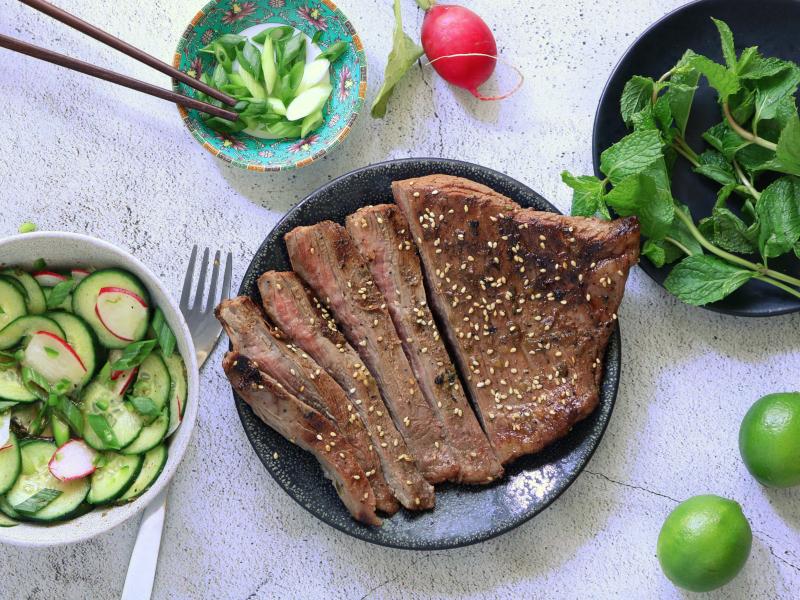This overhead photograph showcases a beautifully plated gourmet meal on a light surface, potentially concrete. Central to the image is a gray plate featuring a medium-rare steak, charred and seasoned with sesame seeds, sliced into four strips with one large uncut piece, revealing a tender pink interior. Adjacent to the steak, on the upper left, lies a single radish. Above the steak is a vibrant bowl filled with greenery, possibly mint, displayed in a floral patterned bowl adorned with purple flowers on a green background. Next to it sits a bowl of green onions, accompanied by chopsticks poised within, suggesting active dining. To the right of the steak is a fork with prongs facing up. Completing the spread, towards the bottom right, are two pristine limes, while to the left of the fork is a bowl of lightly garnished cucumbers and radishes.